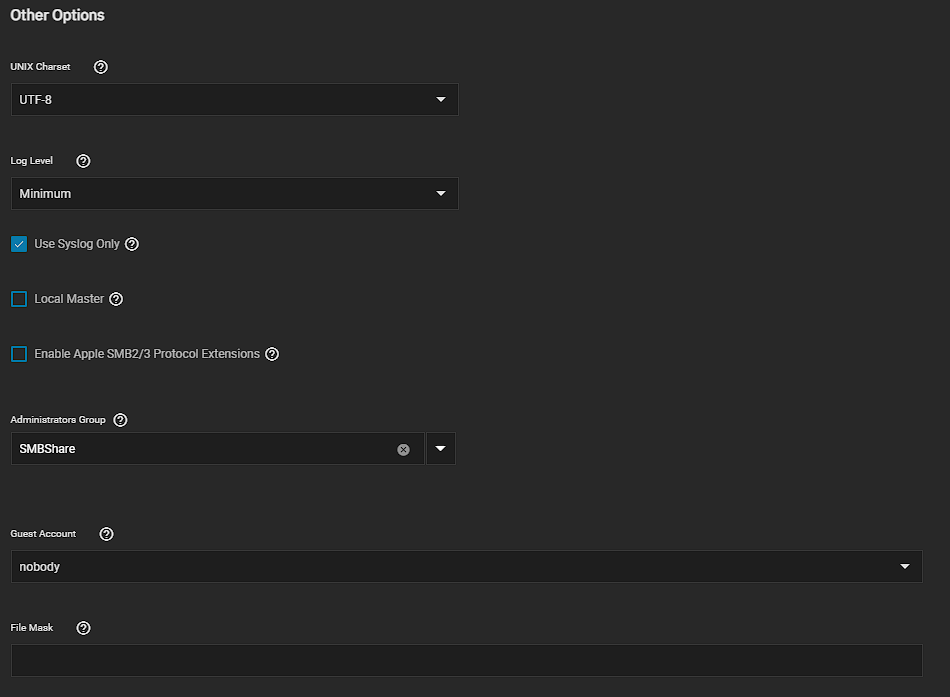This is a detailed horizontal rectangular image featuring white fonts on a predominantly dark background. In the top left corner, the text "Other Options" is displayed in bold white font. Directly underneath, illegible small text is shown next to a white circle containing a question mark.

Below that, there's a darker horizontal rectangle with the text "UTF-8" in all caps, followed by a pull-down menu on the right. Beneath this, in a lighter black area, there's a label that appears to read "Long Level," followed by another darker section labeled "Mont," accompanied by a pull-down menu on the right.

Further down, there are three options, each with a turquoise checkbox to the left. The checkbox next to "Use Syslog Only" is filled in with a white check mark, indicating selection. The other two options, "Local Master" and "Enable Apple SMB2/3 Protocol Extensions," have empty checkboxes.

Towards the bottom, the label "Administration Group" is displayed in small white fonts, followed by the all-caps text "SMB Share Only" to the right with a pull-down menu.

Lastly, the label "Guest Account" appears in white font, followed by the word "nobody" in lowercase in a dark area, with another pull-down menu to its right. The final section labeled "File Mask" is empty.

This image appears to be a configuration or settings interface, possibly for network or file sharing system settings.